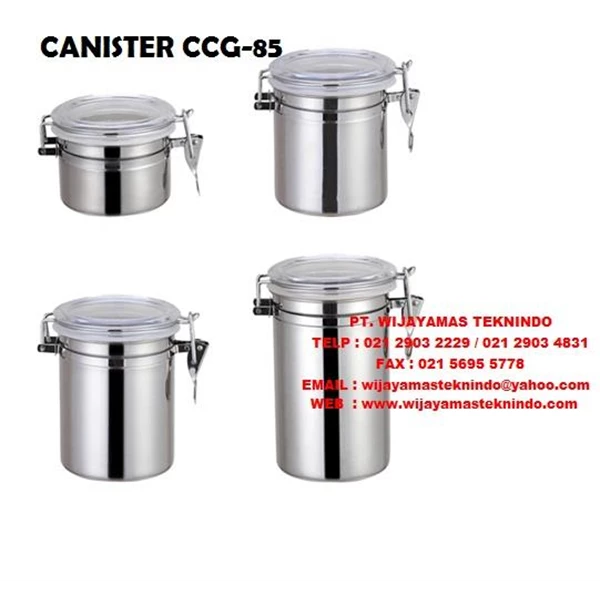The image features four silver metal canisters of varying heights, arranged on a white background. At the top left corner, in black all-capital font, the text reads "CANISTER CCG-85." The upper row contains two canisters, with the one on the left being shorter and wider, having a plastic or glass top with a clasp, and the one on the right being taller and slimmer with a similar design. The lower row features two taller canisters, with the left one being taller than the canisters in the top row, and the right one being the tallest. Each canister has a black stripe running down its center. The lower right-hand canister is overlaid with red text, stating "PT.WIJAYAMAS TECHNINDO" followed by their contact information: telephone numbers "TELP: 021-2903-2229 / 021-2903-4831", fax number "FAX: 021-5695-5778", email "EMAIL: wijayamasteknindo@yahoo.com", and the website "WEB: www.wijayamasteknindo.com".